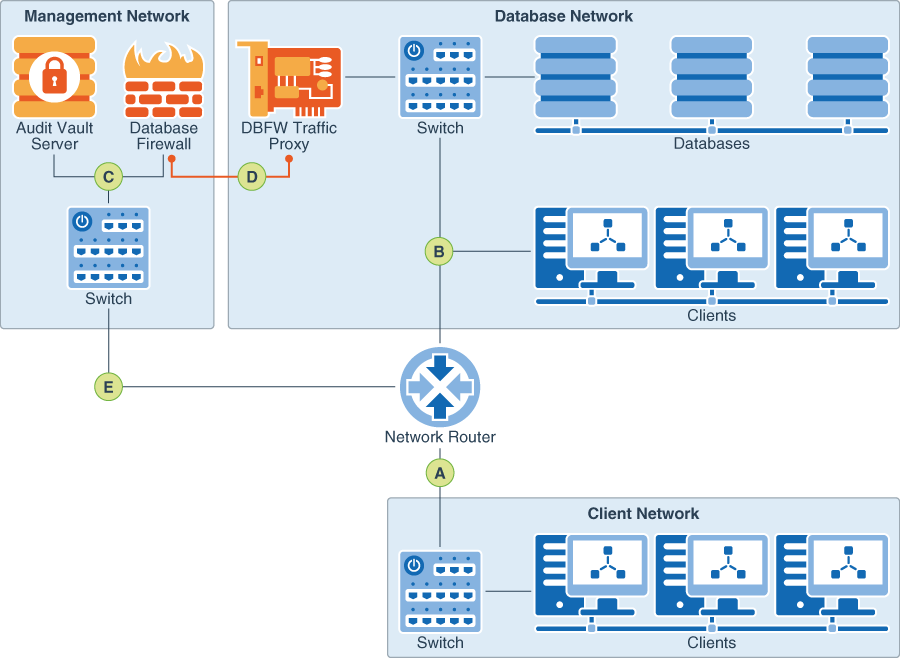The image is a detailed workflow chart with a light blue background divided into three main sections: Management Network (upper left), Database Network (center), and Client Network (bottom). 

In the Management Network section, at the top, there's a bold header labeled "Management Network." Below it, "Audit Vault Server" is indicated, accompanied by an icon resembling a chimney with a lock. Next to it is "Database Firewall," illustrated with bricks and flames. Beneath this, there is a labeled "Switch" with an 'E' underneath.

The central Database Network section, the largest, contains "DBFW Traffic Proxy" in an orange box, followed by "Databases" and "Clients," depicted with three database icons and three animated blue computer monitor icons, respectively. Below, "Network Router" is defined with an icon.

The Client Network section at the bottom consists of a "Switch" and "Clients" labeled next to three animated blue computer monitor icons. Arrows indicate connections between all sections, stemming from the centralized network router, labeled 'A'. 

Overall, the chart visually represents the interconnected Management Network, Database Network, and Client Network, emphasizing the flow and interaction among various network components through directional arrows.